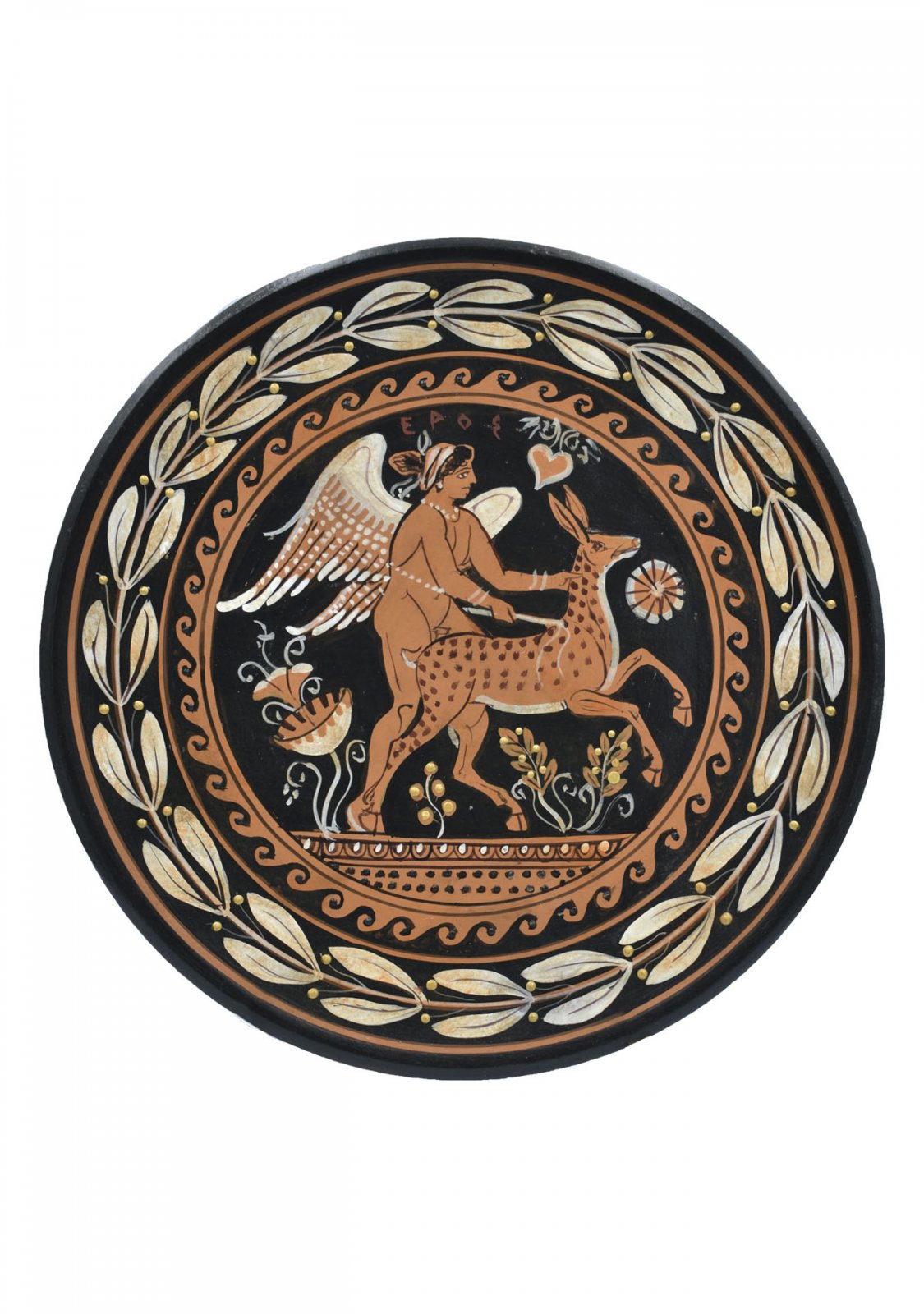This detailed artwork features a central circular image set against a plain white background. The entire piece measures approximately three inches in diameter, with the central, black-bordered circle being about an inch and a half wide. Dominating the inner circle is an intricate scene where a nude male figure with brown skin and white wings, and curly hair, interacts with a spotted deer, characterized by long, bunny-like ears. The man, positioned behind the deer, holds its neck with his left hand, appearing to make an incision between its shoulder blades. This intimate interaction is set against a black background.

Above this central figure, "E-P-O-E" is printed in reddish-pink, with the first 'E' resembling a capital letter and the last 'E' more rounded. To the right of the person and above the deer, a small heart is visible. Beneath them lies a brown walkway decorated with black and white dots, surrounded by what appears to be leaves with berries.

Encircling this central scene, a brown wave-like pattern forms a band around it. Further out, the next layer is a broad black border, followed by a brown ring. Enclosing it all is a white vine woven with white leaves and berries, leading to another brown circle. The outermost edge of the artwork is black, completing the intricate and harmonious design.